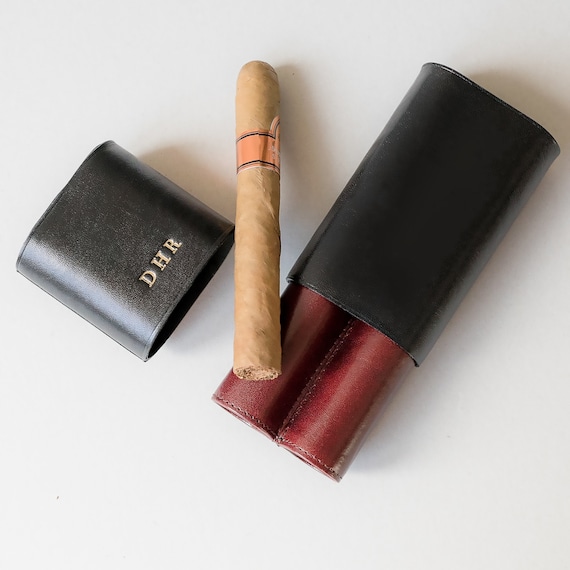The detailed image captures a close-up of a brown cylindrical cigar topped with an orange sticker, placed on a cigar holder. The setting is a light gray flat surface with shadows from the cigar, holder, and lid shifting towards the top right, indicating lighting from the bottom left. The cigar itself displays a rounded end and a flat end, the latter resting partially on the black cigar case. The lid of the case, engraved with gold letters "DHR," lies just to the left of the cigar. The black cigar holder, designed to accommodate two cigars, features two empty red leather-lined compartments. The image, bright and clear, suggests an indoor scene with ample lighting illuminating the arrangement from the bottom left.